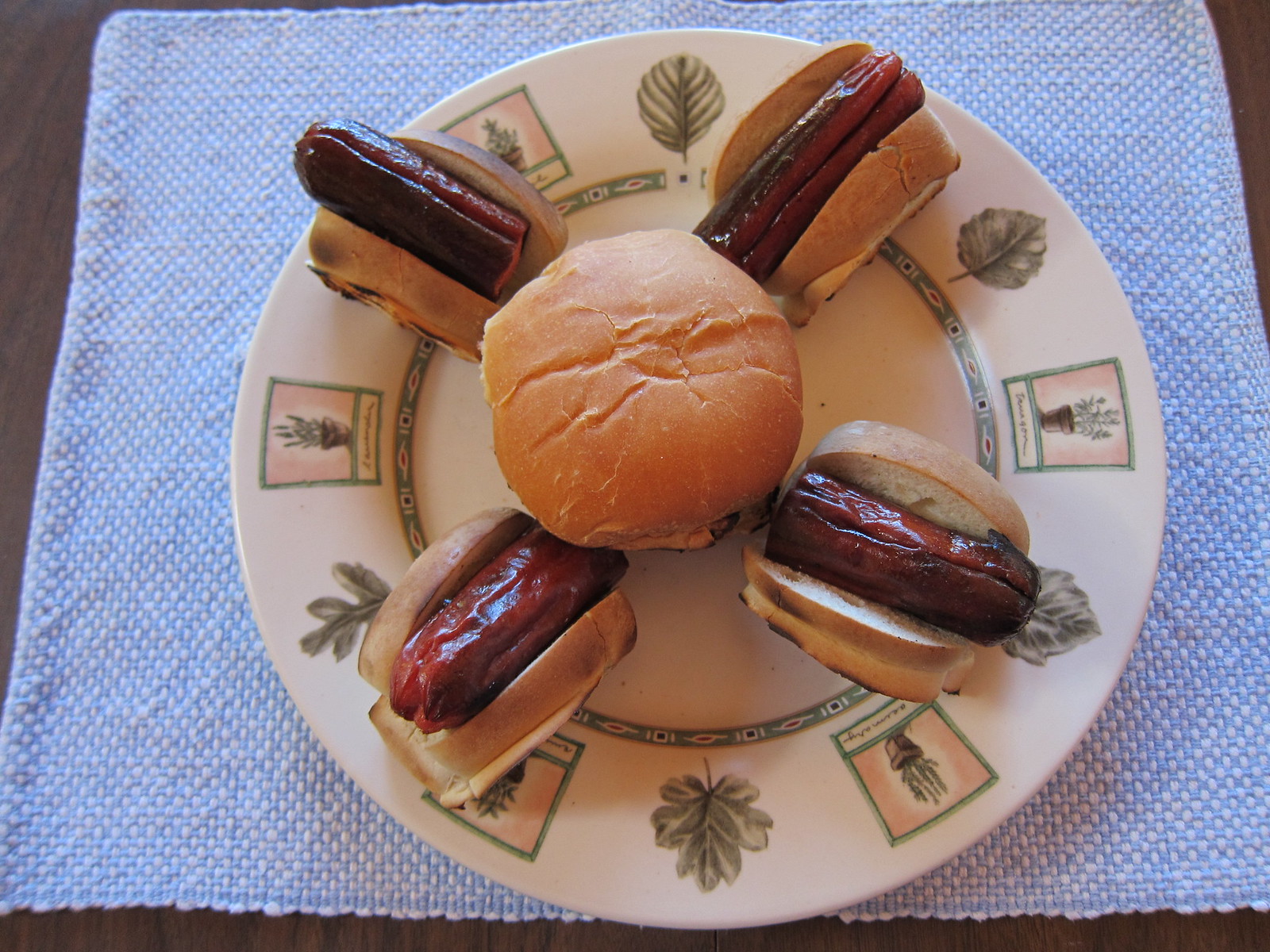In this indoor color photograph, we are looking down at a meticulously arranged plate of food. The centerpiece of the white ceramic plate, adorned with hand-painted green leaves, palm leaves, cacti, and potted plants with black and orange accents, is the top bun of a cheeseburger. Peeking from under the partially broken and bent top bun is a bit of cheese and possibly a hint of the patty itself. Surrounding the central bun are four hot dogs, each split in half and placed in toasted tan dinner rolls, arranged in a spoke-like pattern at approximately the ten o'clock, two o'clock, four o'clock, and seven o'clock positions. The well-cooked sausages display slight blackening and grill marks. The plate rests on a light blue and white checkered kitchen cloth, itself placed on a dark brown wooden table, adding a rustic touch to the scene. The image is well-focused despite the low lighting, emphasizing the intricate details of both the food and the decorative designs on the plate.